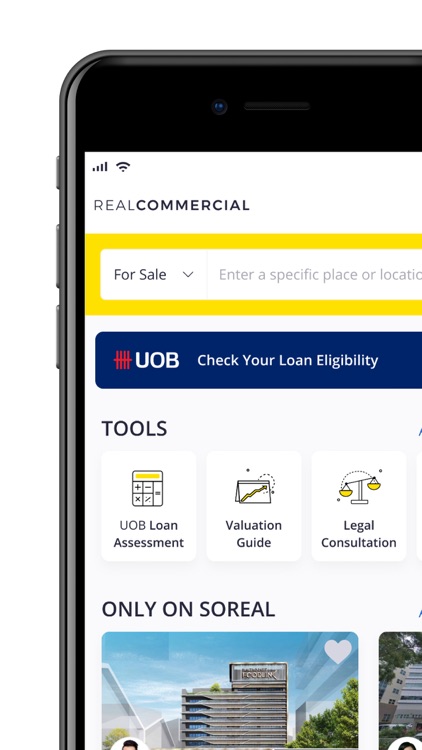This image, captured on a smartphone in a vertical position, shows the left portion of the screen while the right part is cut off. The screen displays a page titled "Real Commercial," with the word "Commercial" prominently bolded in black. Below the title, the phrase "For Sale" appears, followed by an empty space outlined in yellow where one can enter a specific place or location.

Towards the center of the screen, there is a dark blue tab or banner with white text reading "UOB" accompanied by a red logo featuring four or five vertical lines intersected by a horizontal red line. This section prompts the user to "Check Your Loan Eligibility."

Further down, the screen consists of a tools area containing three rectangles, each providing a different description: "UOB Loan Assessment," "Valuation Guide," and "Legal Consultation." Each description is enhanced by a small emblem above it, with the Legal Consultation rectangle displaying a scales of justice icon.

Beneath these tools, in bold black capital letters, the text reads "ONLY ON SURREAL." Below this text, there are two images, one larger than the other, though both are partially cut off. The larger image depicts a blue background with a building in the center, trees at the bottom right, and a white heart in the top right corner.